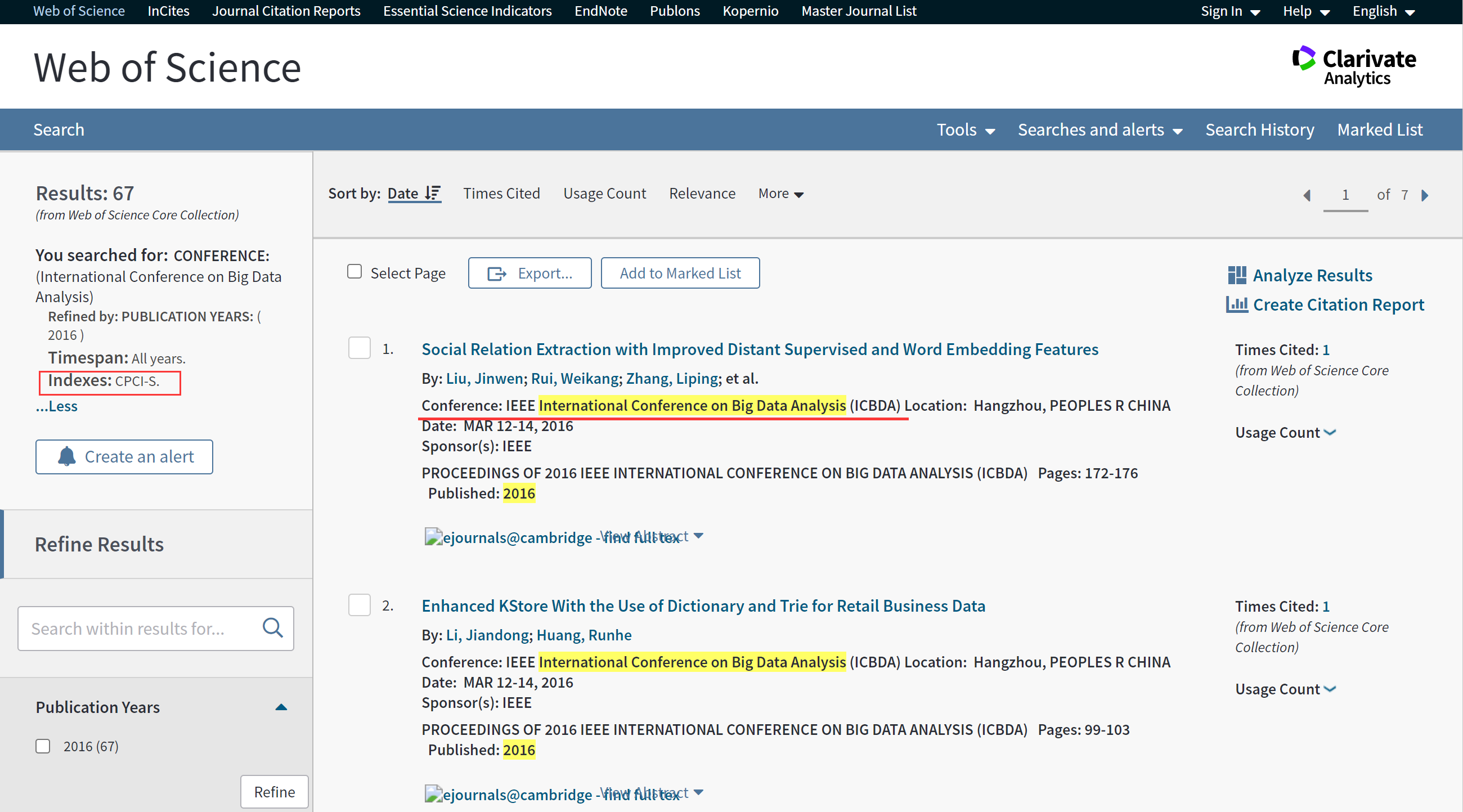The interface of the Web of Science is displayed prominently. The screen's border is black with a blue section on the left, displaying the label "Web of Science" in white text. Adjacent tabs, also stylized in white, denote various sections such as "Insights," "Journal Citation Reports," "Essential Science Indicators," "EndNote," "Publons," "Carbonero," "Nario," and "Master Journalist." At the top right-hand corner of the screen are options for "Sign In," "Help," and language preferences ("English"). A gray background displays "Web of Science" yet again in black text with another tab labeled "Collaborate Analytics" in the right-hand corner.

The banner beneath it features a blue background. On the left side, in white, are the options "Search" and "Tools." The right side of the banner includes "Search and Alerts," "Search History," and "Marked Lists." Below the banner, on the left side in gray, is the label "Results 67," indicating the number of search results from the "Web of Science Core Collection."

A search has been performed for the "International Conference on Big Data Analysis," with results refined by publication years 2016, spanning several years. Highlighted within a red rectangular box, the label "Indexes, CPCI-S" is visible, with options "Less" and "Create an Alert" displayed in blue, followed by "for Refined Results" in black. On the right side, additional filter options labeled "Search by Date" and "Time Cited" are available, though underlined in red, indicating an active selection. 

Highlighted search results include "Social Relation Extraction with Improved Distance Supervised and Word Embedded Features" in blue text. Below, the "Conference IEEE" label is underlined in red, and a specific conference entry, "International Conference on Big Data Analysis (ICBDA)," is highlighted in yellow.